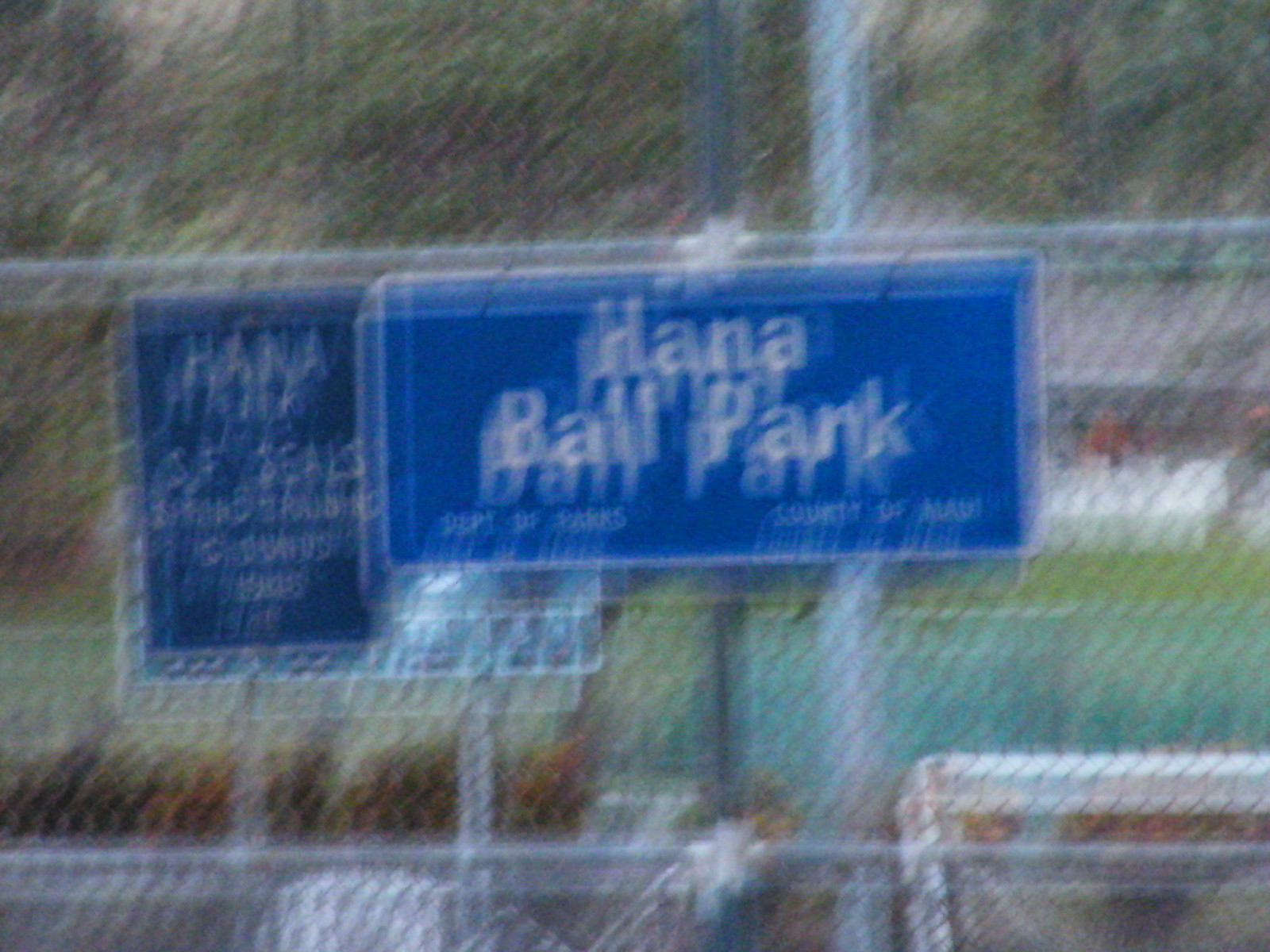The image is a very blurry photograph of a blue rectangular sign mounted on a chain-link fence outside a ballpark. Central to the image, the sign reads "HANA Ballpark" in white letters, although some additional text underneath is too difficult to decipher. Behind and to the left of this sign, there appears to be another blue sign that also features the name "HANA" at the top. The background includes trees, suggesting the ballpark is situated in a leafy area. The lower half of the picture shows the green playing field, possibly a baseball field, with features like benches and what might be bleachers or soccer goals visible through the fence.